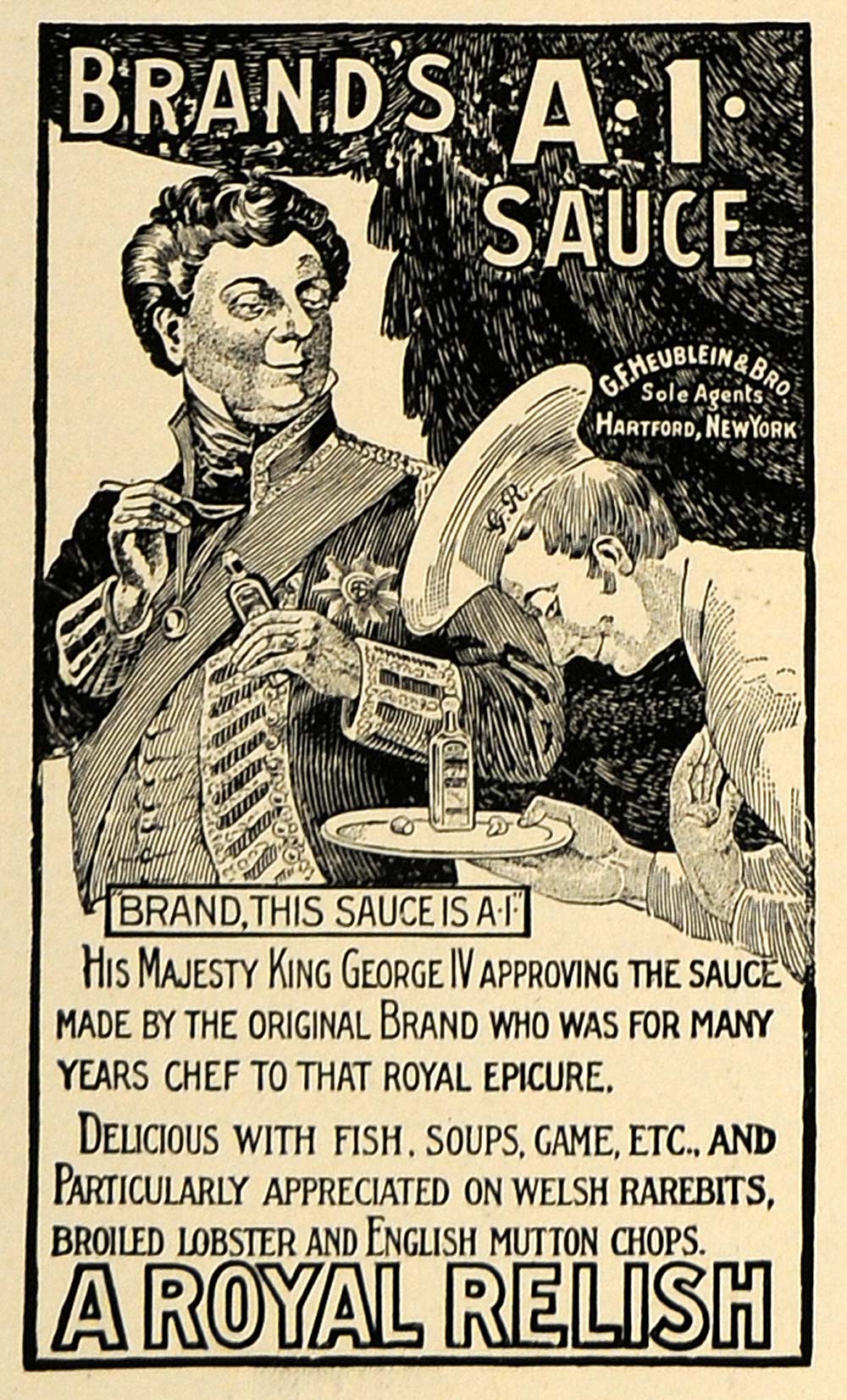This is an antique marketing advertisement for Brand's A1 Sauce, printed on discolored, tan paper that has aged over time. The vintage poster features black ink illustrations and text, with a prominent title at the top stating "Brand's A1 Sauce." The illustration depicts two figures: His Majesty King George IV dressed in regal attire, possibly a soldier or royal prince, and a butler bowing, presenting him a bottle of A1 Sauce on a white platter. A dark curtain hangs over the top of the scene. Beneath the image, the text reads: "His Majesty King George IV approving the sauce made by the original brand who was for many years chef to that royal epicure. Delicious with fish, soups, game, etc., and particularly appreciated on Welsh rarebits, broiled lobster, and English mutton chops—a royal relish." The advertisement is taller than it is wide, enclosed in a black border, with mention of "Sole agents Hartford, New York."